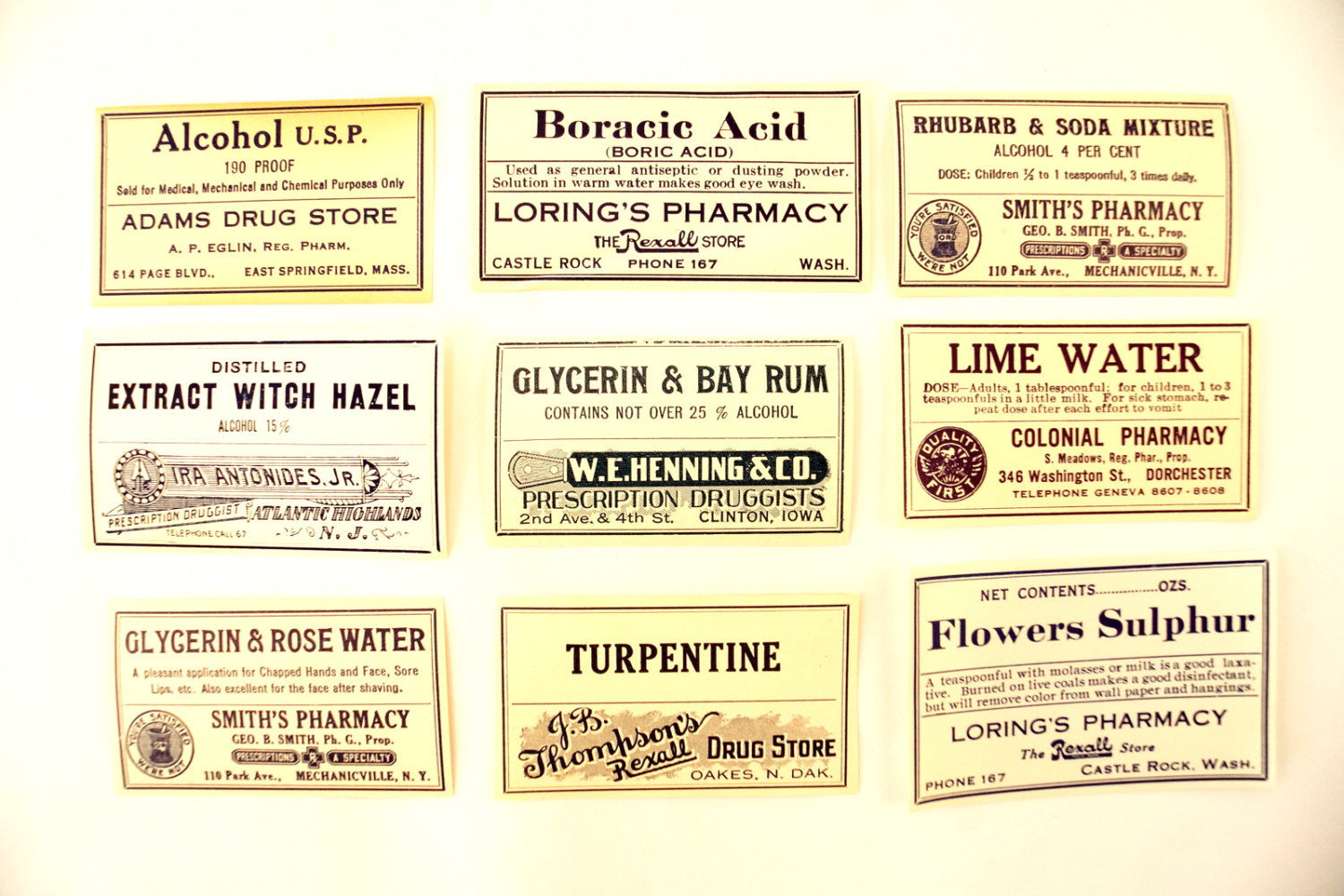The image features nine rectangular labels arranged in three rows and three columns on a background with an aged appearance—off-white, almost pink, with beige-toned corners. Each label represents a different product available at various pharmacies, appearing like vintage advertisements. The products include Alcohol, USP-190 proof from Adams Drugstore, distilled extract Witch Hazel, and Glycerin and Rosewater from Smith's Pharmacy, as well as Boric Acid from Loring Pharmacy, a Rexall store. Additionally, there is Glycerin and Bay Rum available at W.E. Henning and Company, Turpentine from J.B. Thompson Drugstore, Rhubarb and Soda Mixture from Smith's Pharmacy, Limewater from Colonial Pharmacy, and Flowers of Sulfur from Loring Pharmacy. The detailed text on the labels includes information about the uses and instructions for these medicinal and chemical products, such as alcohol being for medical, mechanical, and chemical purposes and boric acid serving as an antiseptic. The labels evoke a nostalgic feeling, possibly being reproductions of original vintage pharmacy advertisements.